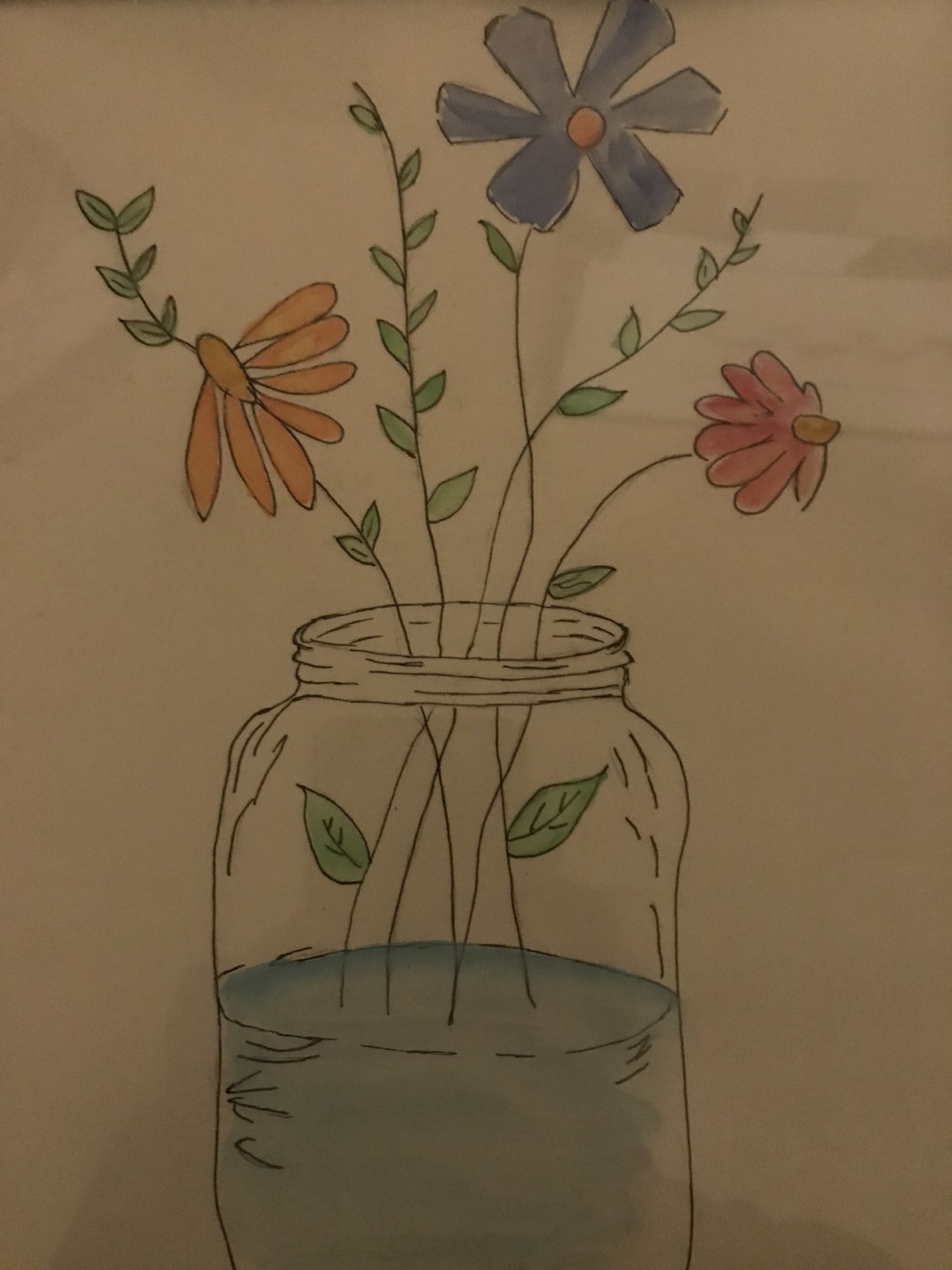This is a color photograph of a watercolor drawing, featured on a white or possibly off-white piece of paper. The drawing depicts a clear glass jar, resembling a mason jar with a screw-on lid that is not attached. The jar is filled halfway with blue water. Emerging from the water are three distinct flowers and several green vines. The left flower is yellow with seven petals, the center flower is blue with six petals arranged in a circular pattern around a yellow center, and the right flower is pink with eight petals facing right, also with a small yellow center. The green vines rise straight up from the water, with two leaves still submerged but extending out from the jar. The detailed pen lines define the jar and vines, while the flowers and leaves are vividly painted with watercolors. The background appears to have a subtle tannish brown hue.